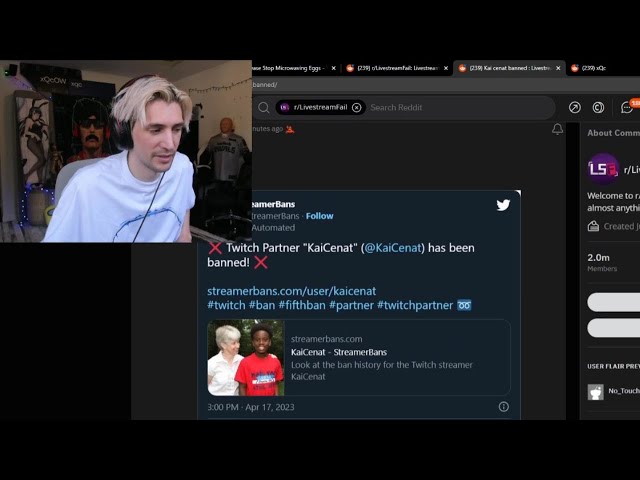The image showcases a computer screen with several elements displayed, primarily in dark mode. The most prominent section features a young man with blonde hair wearing a t-shirt and a pair of headphones. He is situated in a white room adorned with posters. This individual appears to be of European descent and is captured in a small image that occupies the upper left corner of the screen. 

In the background, multiple browser tabs labeled 1, 2, 3, and 4 are visible. These tabs are also in dark mode, with one displaying a screenshot from Twitter. The Twitter interface is in dark mode, highlighted by a white Twitter icon.

At the top of the Twitter screenshot, a red 'X' with white text announces, "Twitch partner Kai Sinat has been banned." Directly below, in sky blue text, there is a URL: "streamerbans.com/user/KaiSinat." Several hashtags underline the message, including #Twitch, #ban, #fifthban, #partner, and #Twitter partner.

Adjacent to the central image, another image features two boys, one of European descent and the other of African descent, though the accompanying text is unreadable. The caption includes "KaiSinatStreamBans" with a timestamp of 3 p.m. and the date April 17, 2023. To the far right of the screen, an information icon is present, adding to the detailed narrative of the scene.